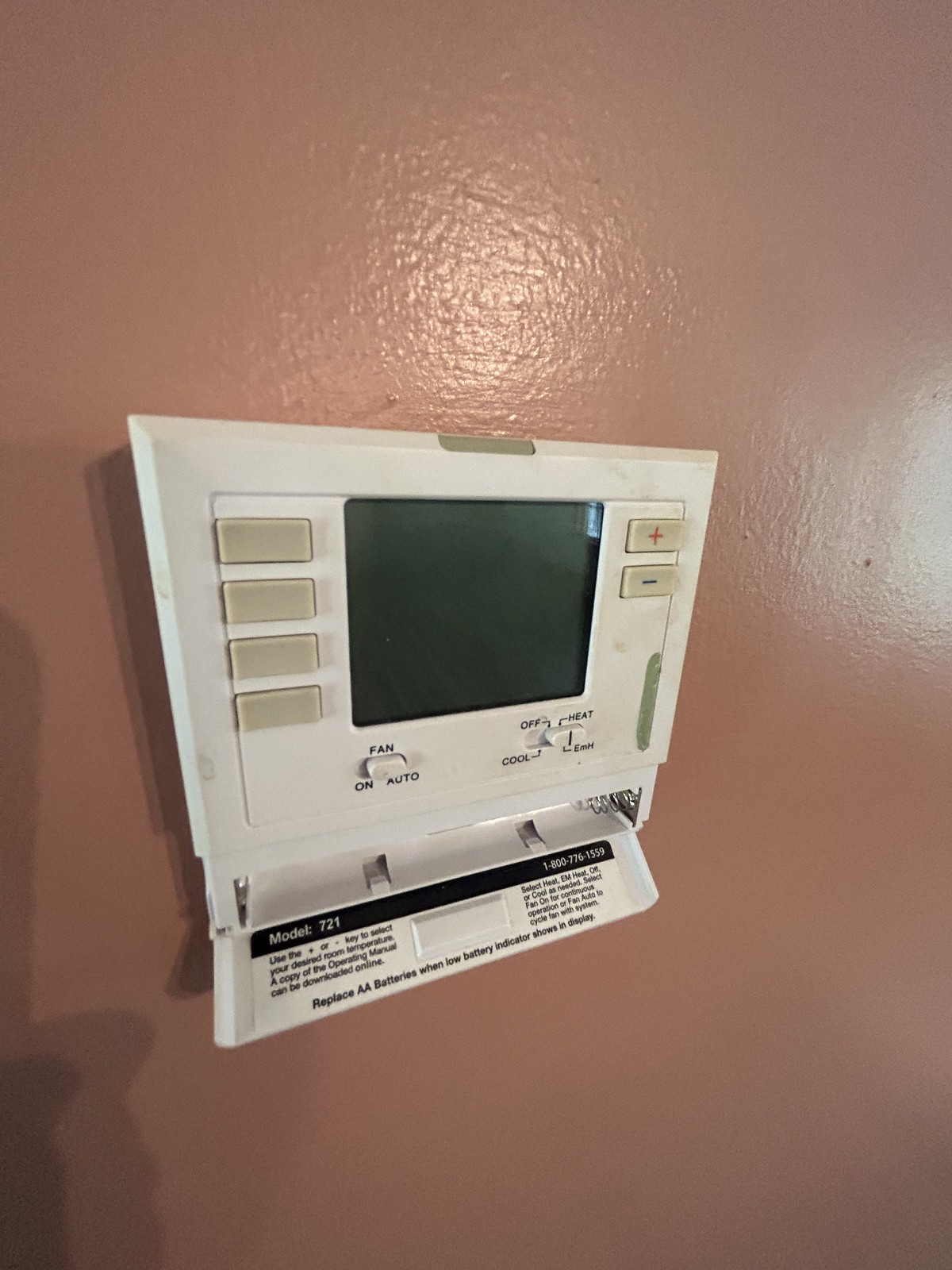Indoor color photograph featuring a slightly distorted view of a peach-painted wall due to a wide-angle lens. Mounted on the wall is an old, rectangular white plastic digital house thermometer, likely from the late 80s or early 90s, showing signs of heavy use and dirt. In the center of the thermometer is a square black LED screen that is turned off, revealing no information.

To the left of the screen is a vertical column of four light grayish-white rectangular buttons. On the right side, two similar rectangular buttons are visible: the upper one marked with a red plus sign and the lower one with a horizontal blue line indicating negative.

Below the display, on the lower left corner, is a fan control switch labeled "Fan," which is moved to the far right within an oval slot. The options "Auto" and "On" are indicated to the left. Correspondingly, on the lower right corner, there is a switch for temperature control, set to "Heat" with "Off" above it, and "Cool" and an illegible label below it.

Additionally, a horizontal battery compartment located beneath the lower center portion of the thermometer is open and empty. Visible inside is a label noting the model number "721," along with some fine print that is too small to read.